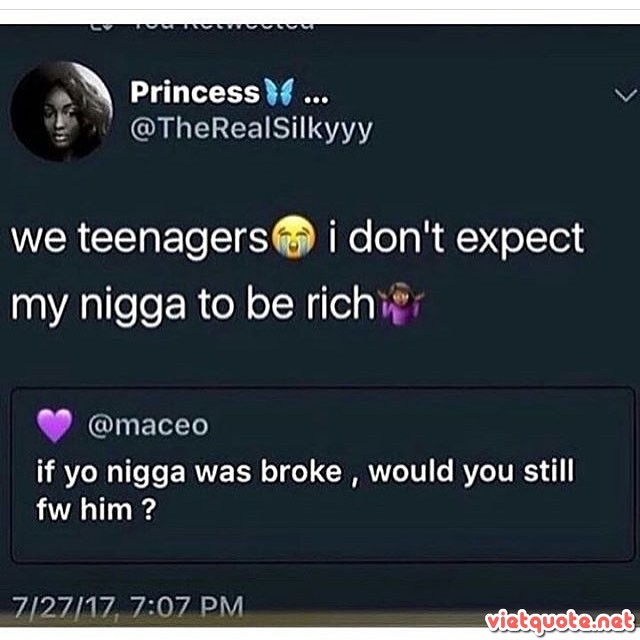The image is a close-up of a tweet from Twitter with a dark brown, gray, and navy blue background. In the top left corner, there's a black-and-white profile picture of an African American girl with medium-length wavy black hair. Beside her picture is the name "princess" followed by a butterfly emoji and three dots, with the handle "@therealsilkyyyy" underneath. The tweet reads: "We teenagers 😢 I don't expect my nigga to be rich 🤷‍♀️." Beneath this, there is a response highlighted in a purple-outlined rectangle. The response, from a user with the handle "@MACE_O" and a purple heart emoji, says: "If yo nigga was broke, would you still F-W with him?" The date and time "7/27/17, 7:07 PM" appear at the bottom left, and in the bottom right, there's red text that reads "via Tquote.net."